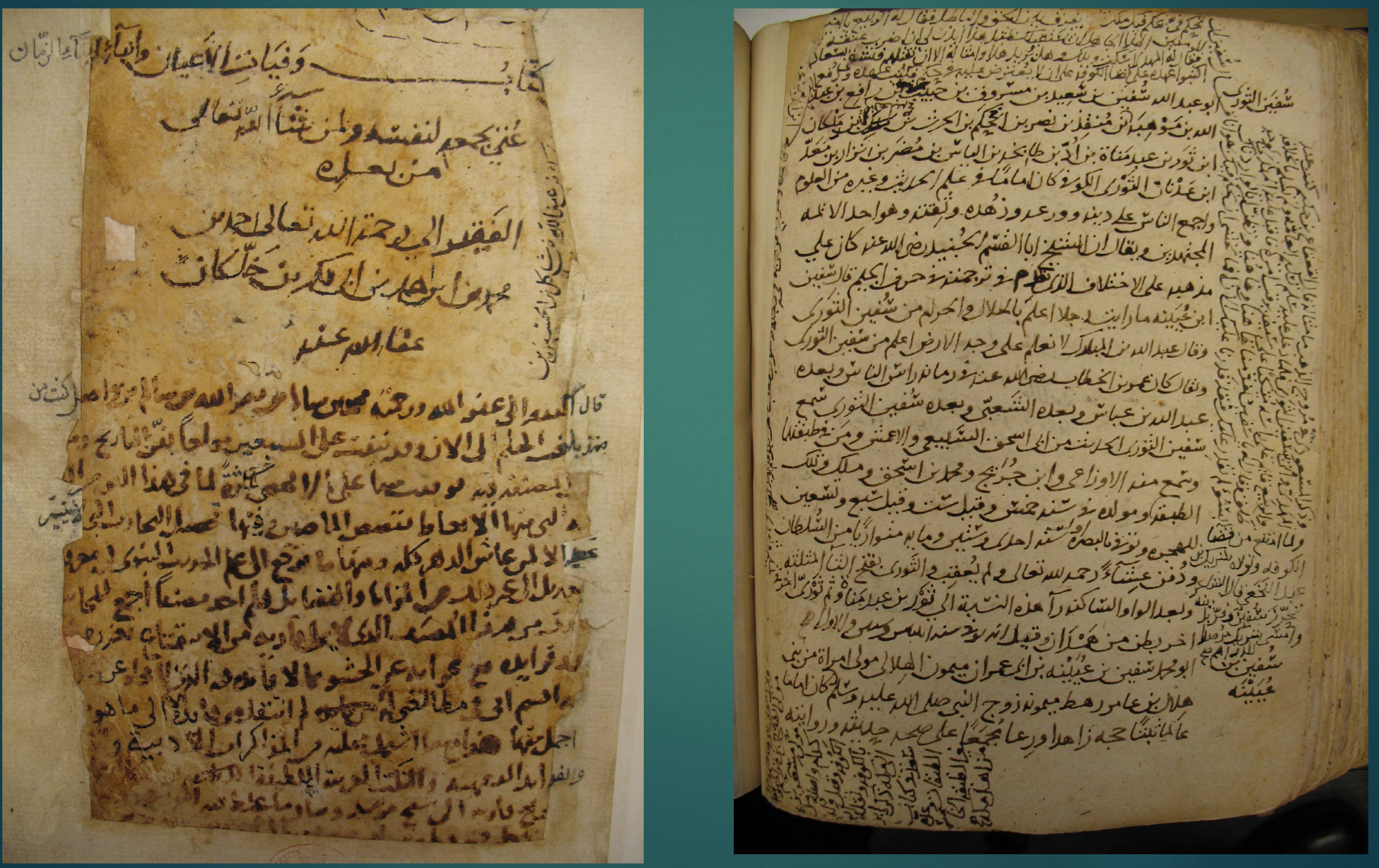The image displays two close-up photographs of an ancient manuscript, oriented horizontally in a rectangular shape. The background is a distinctive teal blue, with a thin vertical bar of the same color dividing the two photos. The left-hand side features a page, showing faint black writing in a foreign language, sparsely populated with text, and appearing as if taken from an old diary or log. The paper reveals signs of age with a rough, worn, and discolored surface, fading from its original white or ivory hue to a very pale yellow. The right-hand side has a denser arrangement of horizontal lines of text, with additional vertical text along the sides and bottom. The manuscript page on the right seems to be part of a thick, open book, as suggested by the visible underlying pages and a black stand beneath. The overall presentation indicates an attempt to preserve and display these fragile, ancient writings.